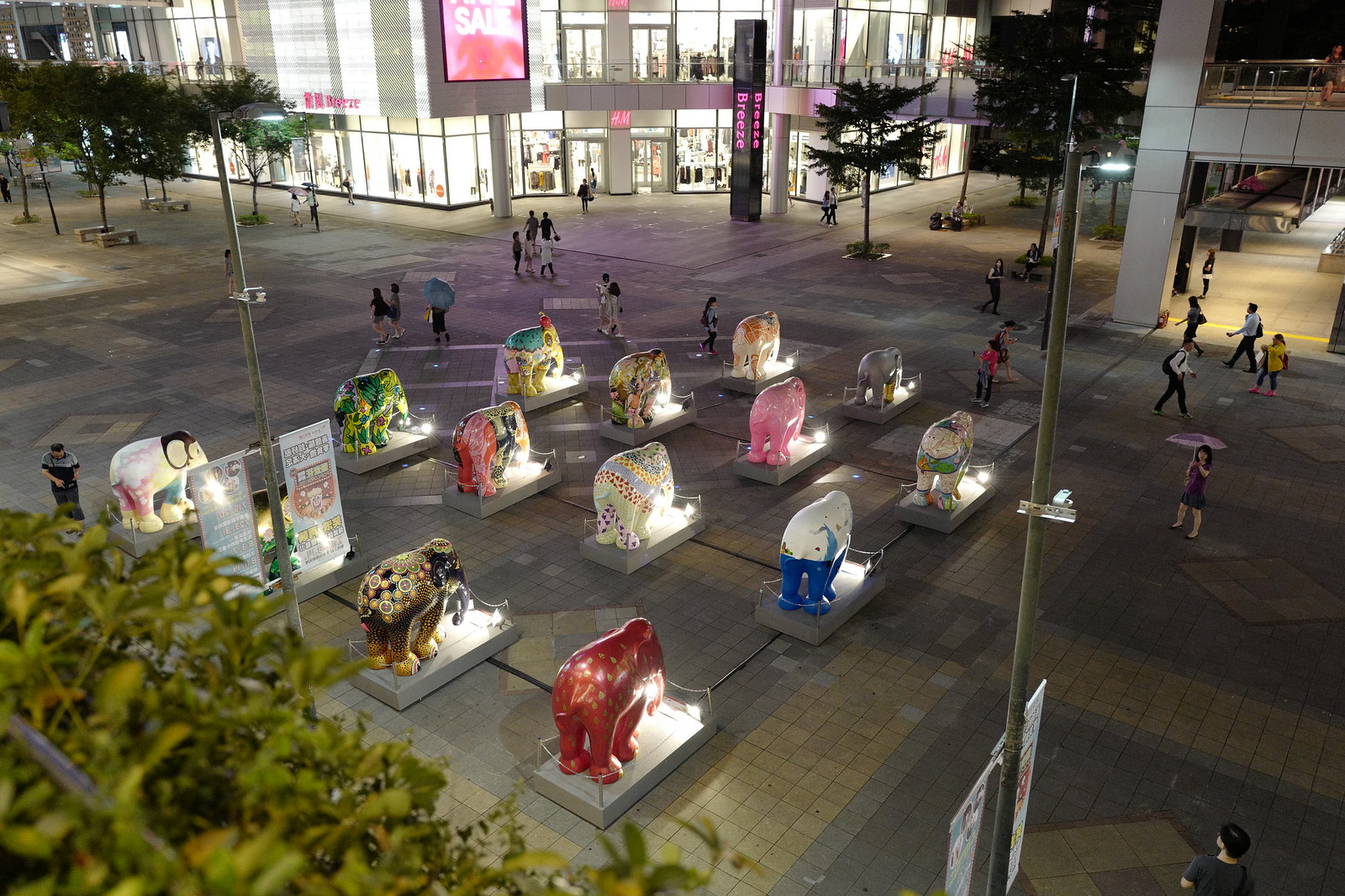This overhead nighttime photograph captures a bustling city square illuminated by bright street lights and shopfront signs, including a prominent "SALE" sign and an H&M logo visible on a two-level mall. The main feature of the square is an eye-catching art installation of 14 brightly colored elephant sculptures, arranged in a 4x3 grid with two additional elephants at the front. Each elephant, mounted on rectangular white bases, is uniquely painted in vivid designs—ranging from solid red and pink to intricate patterns of blue and white—suggesting individual contributions from community members or various artists. People, some holding umbrellas, stroll through the square, which is void of cars and adorned with trees and foliage, adding to the lively yet serene atmosphere. The vantage point from a higher location, possibly a balcony or parking structure, provides a comprehensive view of this dynamic urban tableau.